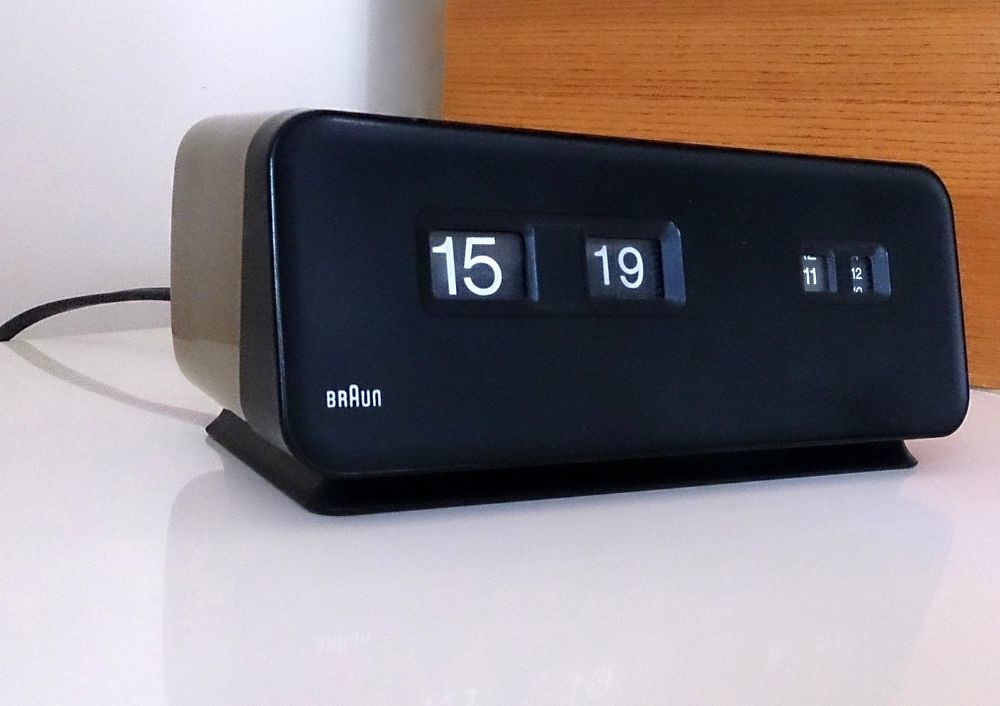This detailed close-up image showcases a Braun digital bedside clock, a blend of sleek design and functional elegance. The clock features a prominent black front panel with an elongated, oval-shaped top, delivering a modern aesthetic. Encased in a sophisticated gray housing, the clock stands on a flat base, ensuring stability on your nightstand. On the right side of the clock, a smaller display highlights the numbers '11' and '12', possibly indicating the alarm or other functional settings. Dominating the center of the clock is a large digital display showing the time as 15:19, underscoring its primary purpose of timekeeping with clarity and precision.